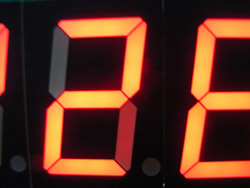The image depicts a black gauge or clock, likely of an analog system. The clock face features numbers glowing in a neon orange color, providing a striking contrast against the dark background. The numbers are designed to appear as though they are cut out from the dark background and illuminated with a lighter gray inside. In the center of the image, the number "2" is prominently displayed, with the upper portion in gray and the lower portion in deep red, adding to the analog aesthetic. Adjacent to the "2," the number "8" is also clearly visible. To the left of these numbers, there's another digit, though its details are indistinguishable. The distinct coloration and design suggest the use of specialized lighting technology typical in analog systems.